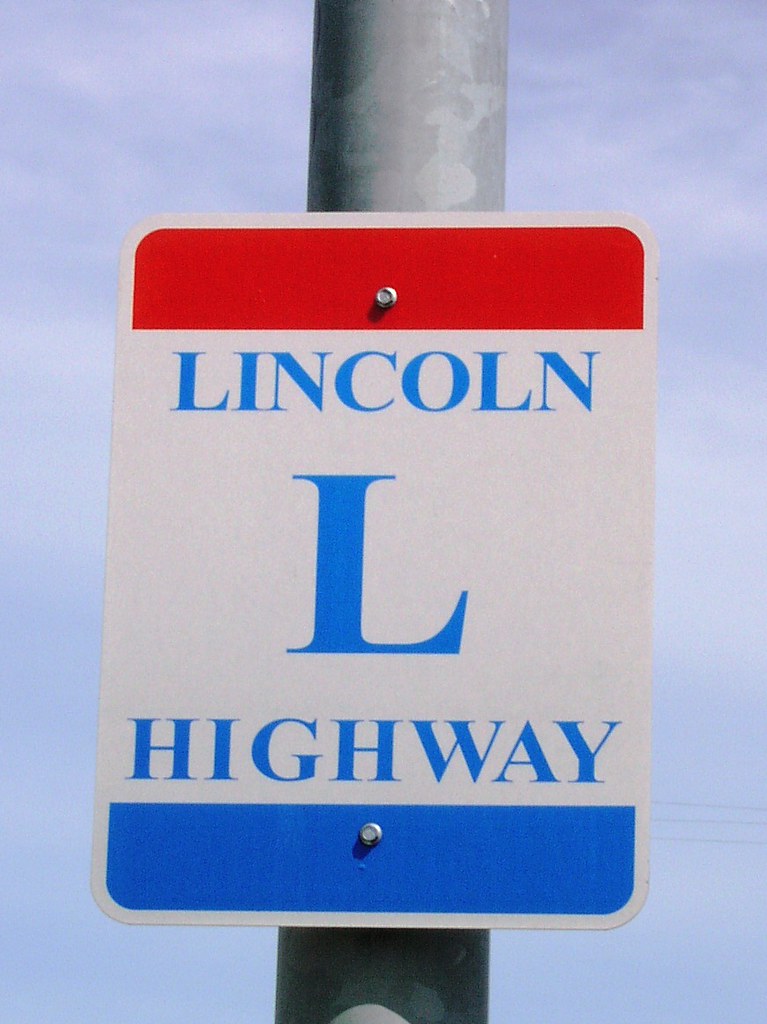A white sign mounted on a gray galvanized steel pole is prominently featured. The sign has a red banner across the top and a blue banner across the bottom. Between these banners, in bold blue letters, it reads "LINCOLN HIGHWAY," with the word "LINCOLN" in all caps and "HIGHWAY" in smaller uppercase letters. At the center of the sign, where the red and blue banners meet, is a noticeable silver bolt, securing the sign to the pole. The pole itself has a unique camouflage pattern, displaying three different shades of gray, resulting from the galvanization process used to prevent rust. The background of the image consists of a cloudy sky with patches of blue peeking through.